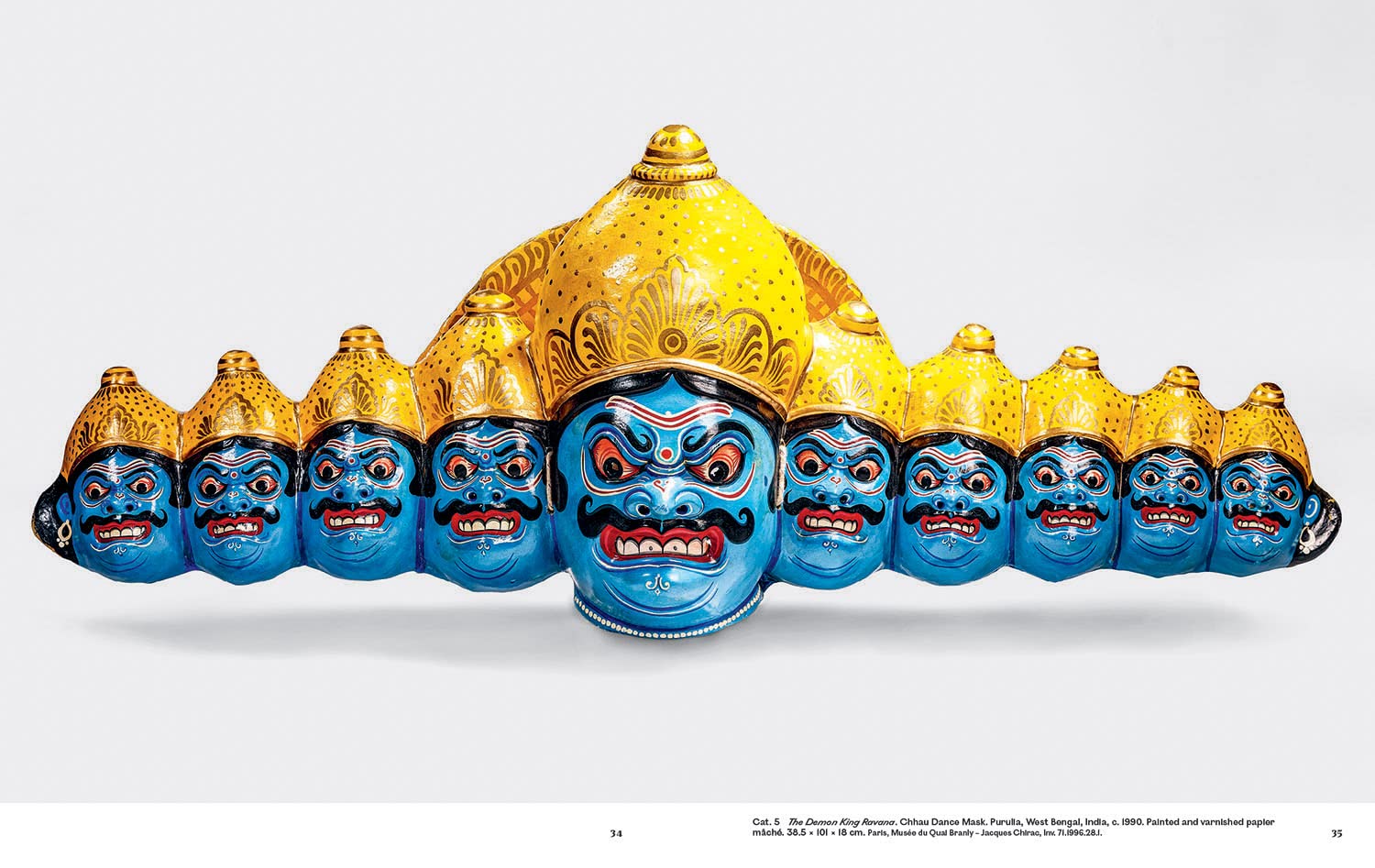The image features a vividly detailed depiction of a mythological Indian figure known as "The Demon King," deriving from the Chichua Dance Mask tradition of West Berlingo, India, circa 1990. The central element is a large, blue-painted head with distinct, demonic features: furious red eyes, curvy black eyebrows, a squiggly mustache, and an open red mouth exposing sharp white teeth. The head bears a golden, Aladdin-style, dome-shaped cap adorned with intricate floral designs and golden dots, reflecting light brilliantly.

Framing this central figure, there are nine smaller, similarly styled blue heads—five on the right and four on the left—all arranged to form a crown-like structure. Each of these heads mirrors the menacing expression of the main head, characterized by their angry, red-highlighted eyes and facial contours, deeply etched lines on the forehead and beneath the eyes, and faint black hair tucked under their golden caps. The background of the image is a subtle grey, with a discernible drop shadow adding depth to the composition. In the bottom right-hand corner, a small print details the artwork’s title and origin: "The Demon King," Bravia, Chichua Dance Mask, West Berlingo, India, 1990, painted and varnished, Pallader.